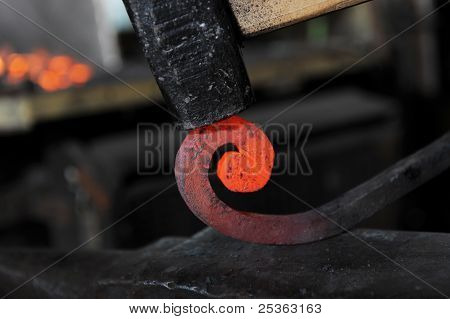The stock image depicts an intense blacksmithing scene, identifiable by the watermark "Big Stock" with an "X" across the middle and the identifier www.bigstock.com 25363163. Central to the composition is a black mallet with a brown handle, poised to strike a glowing piece of metal atop an anvil. The metal, bright orange at the tip from the heat, gradually darkens to black as it curls into a spiral shape. The background is intentionally blurred, with out-of-focus bright lights suggesting high temperatures typically associated with a blacksmith’s workspace. The illuminated workspace adds to the ambiance, emphasizing the focus on the heated metal and the precision of the blacksmith’s craft.